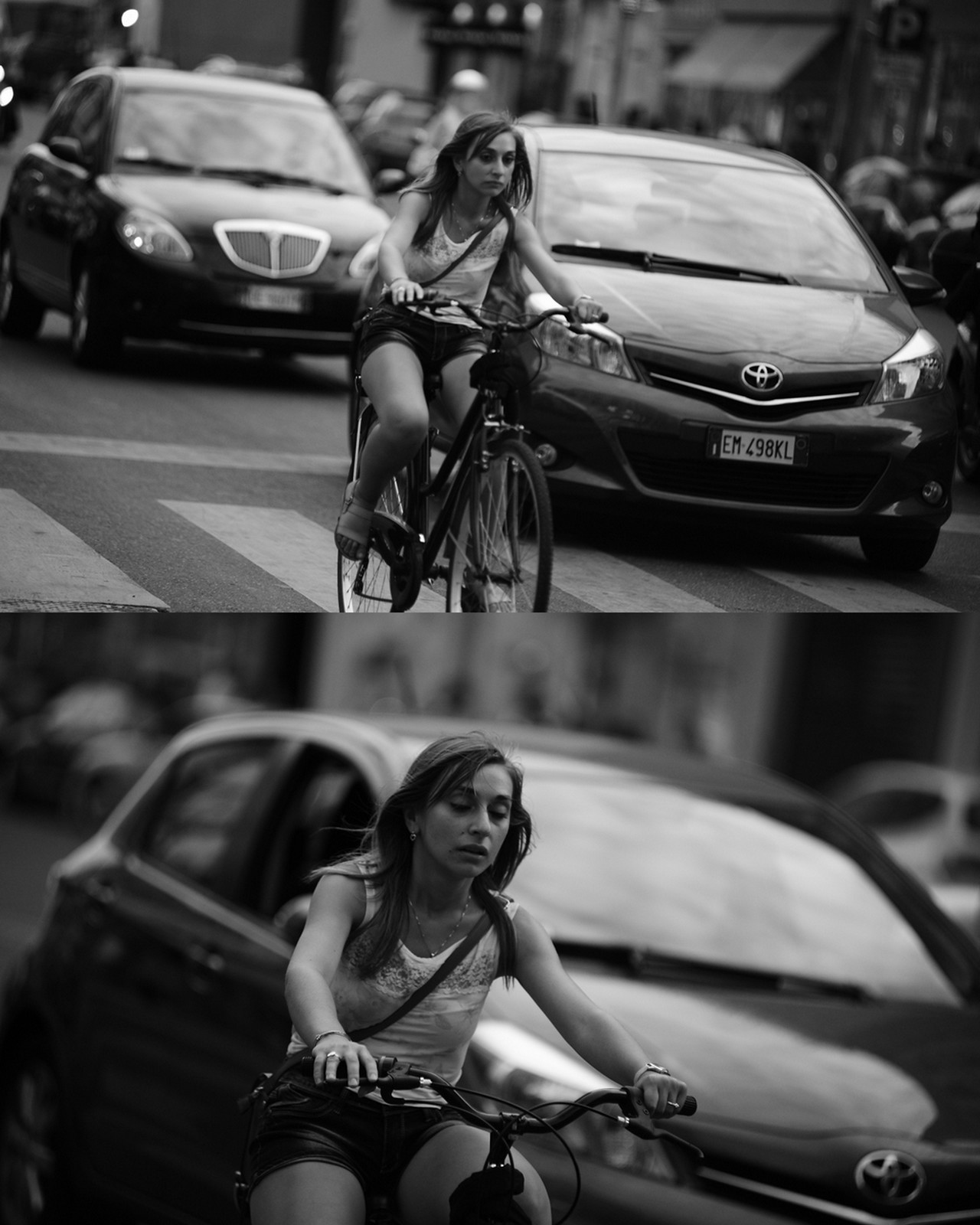This image features a collage of two vertically aligned black-and-white photographs of a city street. Both shots emphasize a medium-skinned girl with long, straight dark hair, as she rides a black bicycle across a crosswalk. In the top photograph, she is captured from a distance, wearing a white tank top, dark shorts, and light-colored flat shoes. Her hands grip the handlebars, and her feet are on the pedals. Two black sedans drive closely behind her, and further back, pedestrians walk along the bustling sidewalks with tall buildings framing the scene.

The bottom photograph provides a closer view of the same scene, zooming in on the girl and capturing more details. Her expression is different here; she looks down, and her eyes appear almost closed, perhaps to avoid the camera. The close-up reveals additional accessories: a watch on her left wrist, a ring on the third finger of her right hand, a cap on her head, and a handbag slung over her left shoulder. Only one of the sedans remains visible in this shot, focusing more intensely on her altered posture and facial expression.